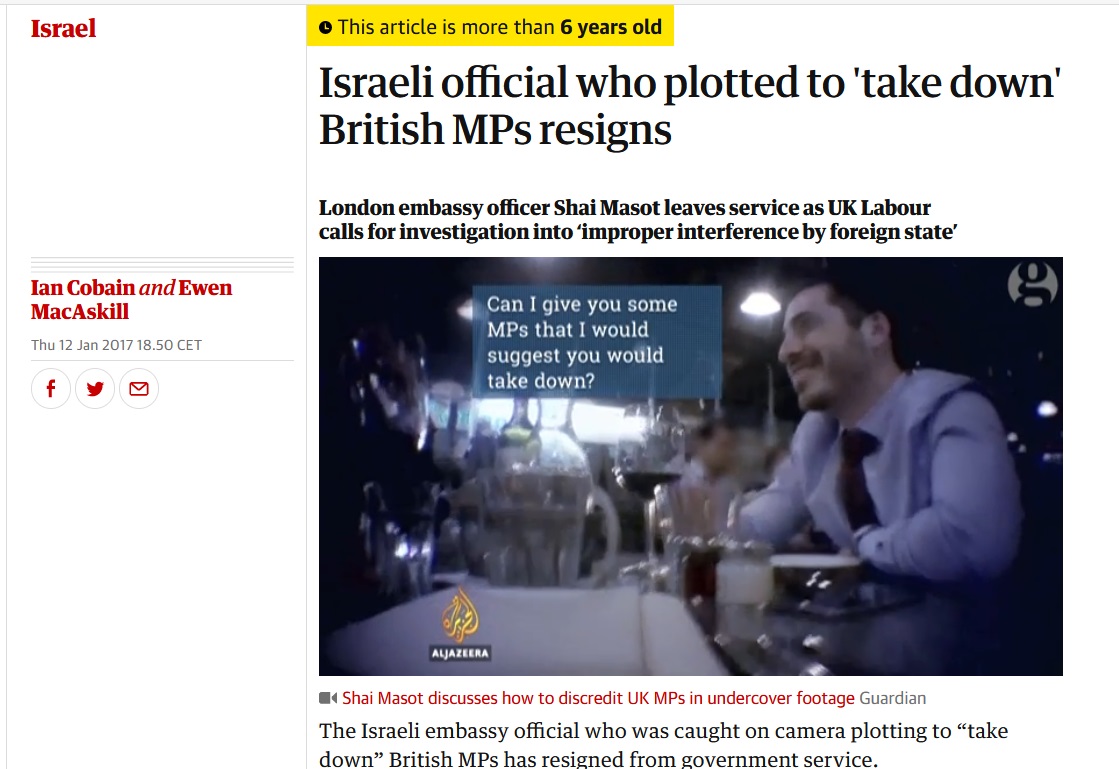**Screenshot of a News Article:**

At the top of the screenshot, a label highlights that the article is over six years old. In the top left corner, the word "Israel" is prominently displayed, indicating the section of the website. A column on the left-hand side lists the authors, Ian Cobain and Ewan MacAskill, and the publication date, Thursday, 12th January 2017.

The headline reads: "Israeli official who plotted to take down British MPs resigns. London Embassy officer Shai Massot leaves service as UK Labour calls for investigation into improper interference by foreign state."

Below the headline, there is an image of a smiling man, Shai Massot, looking to his left. He appears to be in a bar or restaurant, sitting at a table, wearing a light blue button-up collared shirt and a tie. Other patrons are visible in the background. Overlaying the middle of the image, a blue box showcases a shocking quote: "Can I give you some MPs that I would suggest you would take down?"

Beneath the image, a caption reads: "Shai Massot discusses how to discredit UK MPs in undercover footage." The accompanying text explains that the Israeli embassy official, caught on camera plotting to discredit British MPs, has resigned from government service.